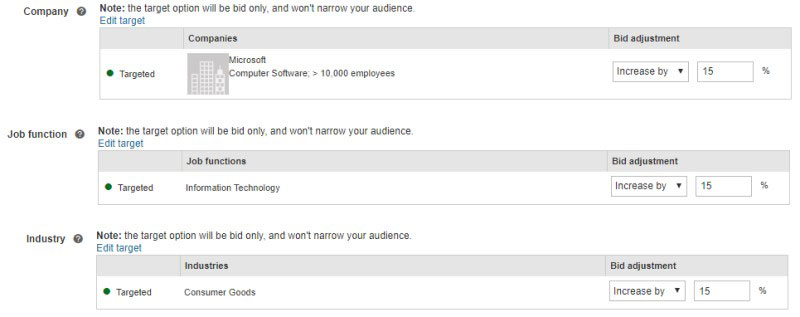The image depicts a section of a webpage dedicated to managing advertising settings. The layout is organized into three rectangular sections, each corresponding to different targeting criteria: Company, Job Function, and Industry. At the top of each section, there is a note explaining that the "target option will be bid only and won't narrow your audience," accompanied by a circled question mark icon labeled "Note." Each section also features an "Edit Target" link. 

Within each rectangle, a green dot signifies that the criteria (Company, Job Function, and Industry) are targeted. All three sections display the same bid adjustment details, stating "increased by 15%". Specifically, the Job Function section highlights "Information Technology," whereas the Industry section mentions "Consumer Goods". 

This well-structured interface appears to assist users in finely tuning their advertising strategies without limiting the audience scope, providing clear instructions and easy access to edit options.